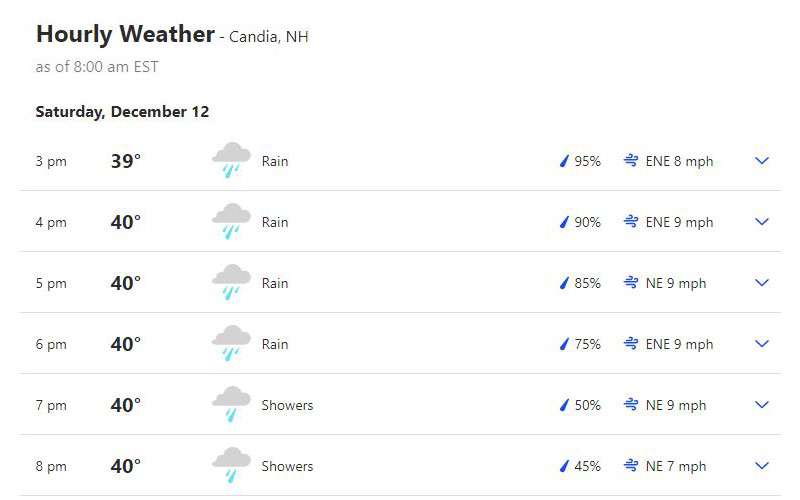Caption: 

The image provides a detailed hourly weather forecast for Kandia, Asia, as of 8:00 a.m. EST, Saturday, December 12th, against a white background. The text is in black, with the header "Hourly Weather - Kandia, Asia" positioned at the top left corner. Various weather icons, including clouds with blue droplets, represent different precipitation levels and occurrences. Key weather details are outlined as follows:

- **3:00 p.m.:** Temperature: 39°F, Rain: 95% chance, Wind: 8 mph East-Northeast.
- **4:00 p.m.:** Temperature: 40°F, Rain: 90% chance, Wind: 9 mph East-Northeast.
- **5:00 p.m.:** Temperature: 40°F, Rain: 85% chance, Wind: 9 mph East.
- **6:00 p.m.:** Temperature: 40°F, Rain: 75% chance, Wind: 9 mph East-Northeast.
- **7:00 p.m.:** Temperature: 40°F, Showers: 50% chance, Wind: 9 mph East.
- **8:00 p.m.:** Temperature: 40°F, Showers: 45% chance, Wind: 7 mph East.

The drop menu for each hour is marked in blue, synchronized with blue precipitation and wind speed icons, illustrating a visually cohesive and detailed weather report.